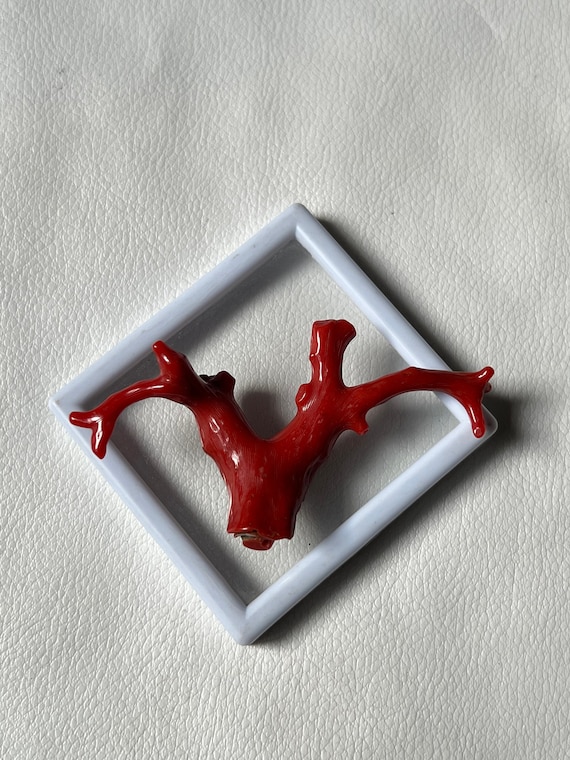The image depicts a vertical, rectangular photo with a textured, white leather background, resembling a car seat. At the center of the image is a glossy white square, oriented at a 45-degree angle, giving it the appearance of a diamond shape. Overlaid on this diamond-shaped square is a striking, deep red, glossy formation that resembles deer antlers or a branching artery system, extending from the left corner, dipping in the center, and connecting to the right corner. This organic, sculpture-like structure stands out vividly against the minimalist and monochromatic background, creating a visually intense focal point.